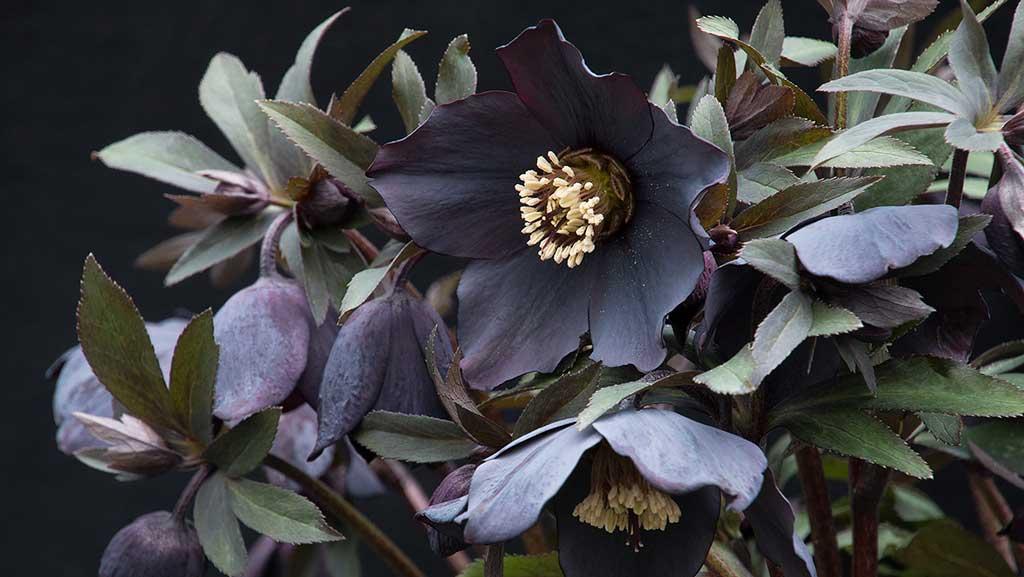The image beautifully captures a type of rose known as Helleborus with a deep gothic appeal. The flowers, appearing almost black, are a blend of deep, dark purple and crimson, striking against the nearly pitch-black background. The focus is on a couple of the flowers in the bush, one flower pointed downward and another facing at a slightly oblique angle. The leaves, deep green with subtle undertones of the same dark purple-red tinge, add to the brooding atmosphere. One of the prominent flowers displays a cluster of yellow pollen in its center, which contrasts sharply with the dark petals. Each flower appears to have five thick, indigo-shaded petals, while the jagged-edged leaves further enhance the dramatic scene. The professional lighting and high contrast successfully evoke a very gloomy, almost surreal and artificial vibe, emphasizing the rich textures and colors of the flowers and leaves.